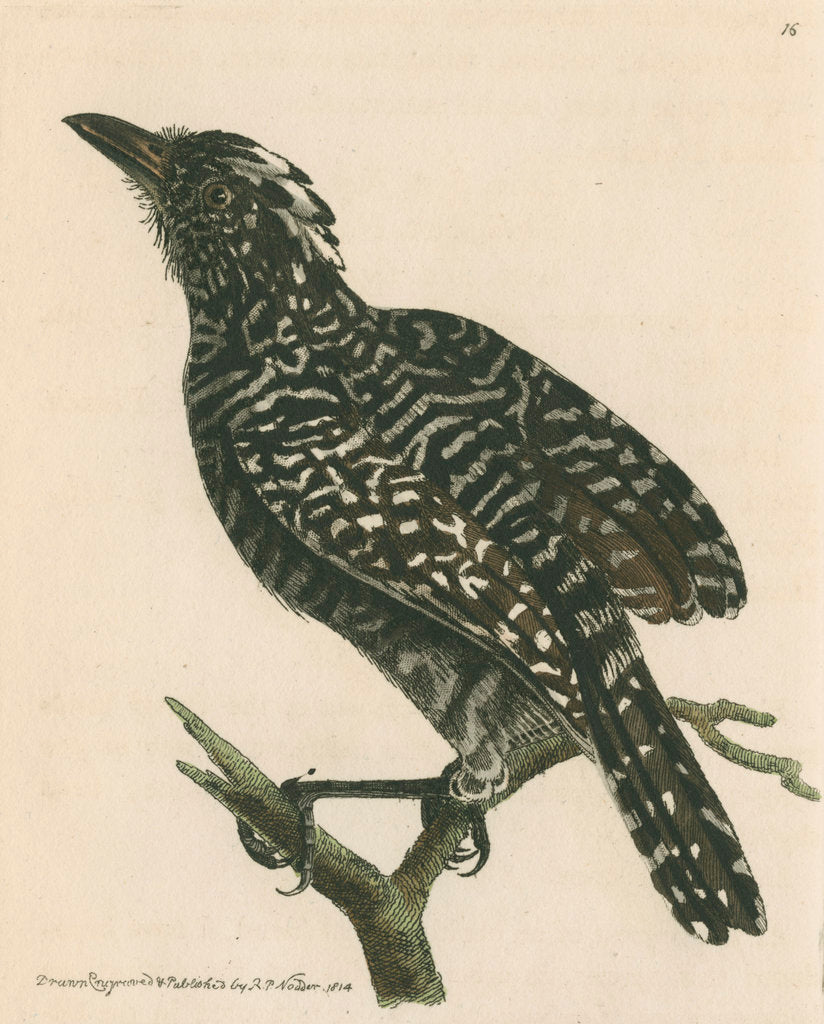This image is a detailed drawing of a bird perched on a Y-shaped branch. The bird, resembling a black crow, has a striking black and gray speckled pattern throughout its feathers, which look meticulously shaded. Its black beak features hints of brown and dirty yellow, complementing its eyes that are a deep black with a gold ring around them. The bird's legs and claws are also black with long nails, gripping onto the intricately detailed branch. The background is a pale tan or camel color, adding a subtle contrast to the monochrome bird. The top right corner bears the number 16, and there is script-like writing at the bottom left, though it's too small to decipher clearly.